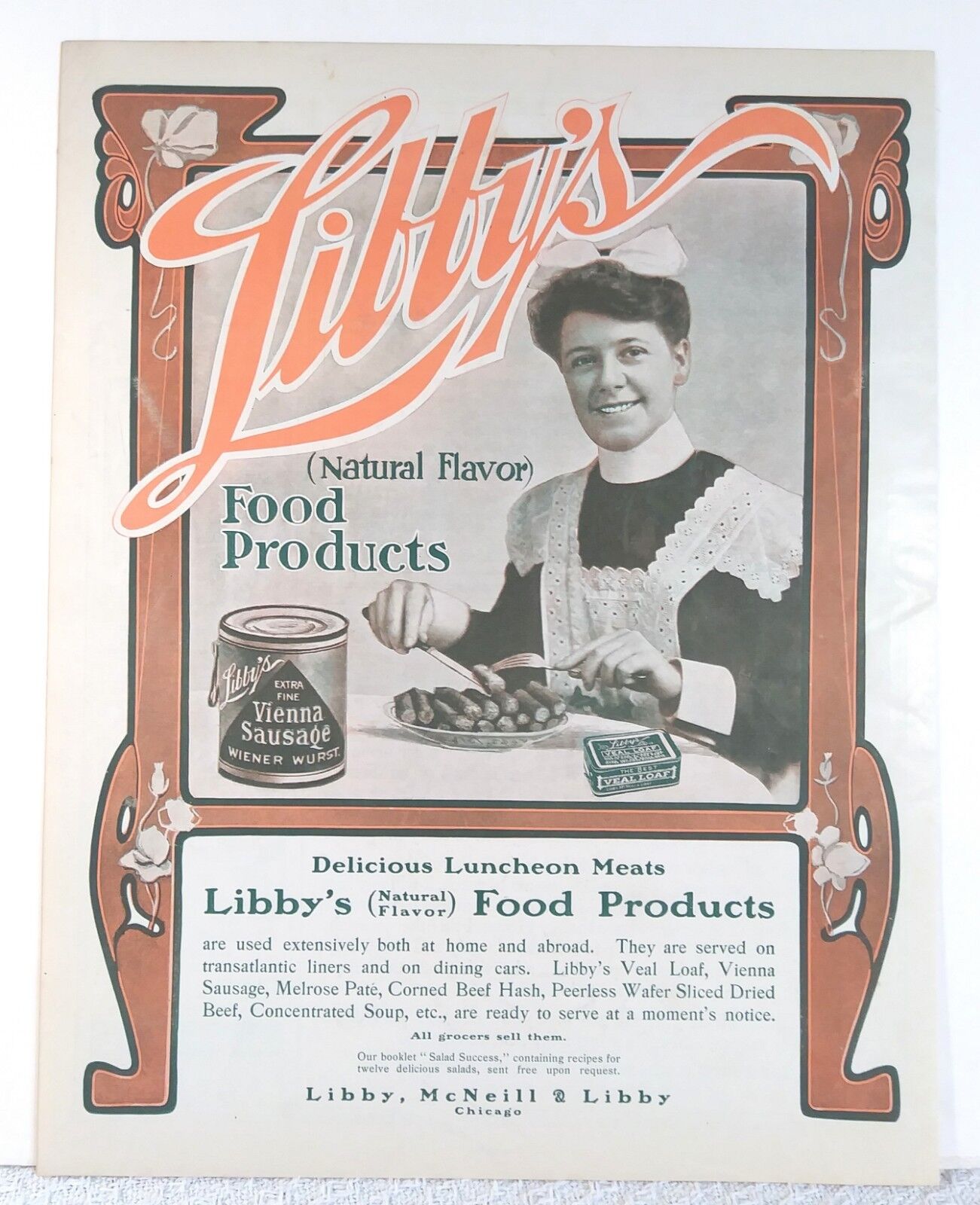The image depicts an old-fashioned magazine advertisement, likely around 75 years old, for Libby's food products. The ad features a slightly yellowed, off-white background with a brownish-orange frame. In the upper left corner, the name "Libby's" is written in a cursive, peach-colored font. At the center, a black-and-white photograph showcases a woman in her 30s with short brown hair, dressed in a traditional maid's outfit—black with a white apron and a white bow in her hair. She is depicted cutting into a plate of Vienna sausages, with a can of "Libby's Extra Fine Vienna Sausage - Wienerwurst" visible to her left.

A detailed paragraph at the bottom of the frame describes Libby's range of delicious luncheon meats, emphasizing their natural flavor and widespread use both at home and abroad, including on transatlantic liners and dining cars. The text lists various other Libby’s products such as veal loaf, Melrose Pate, Corned Beef Hash, Peerless Water Sliced Dried Beef, and Concentrated Soup, all ready to serve instantly. The advertisement also mentions a free recipe booklet titled "Salad Success" available upon request from Libby, McNeil, and Libby of Chicago.